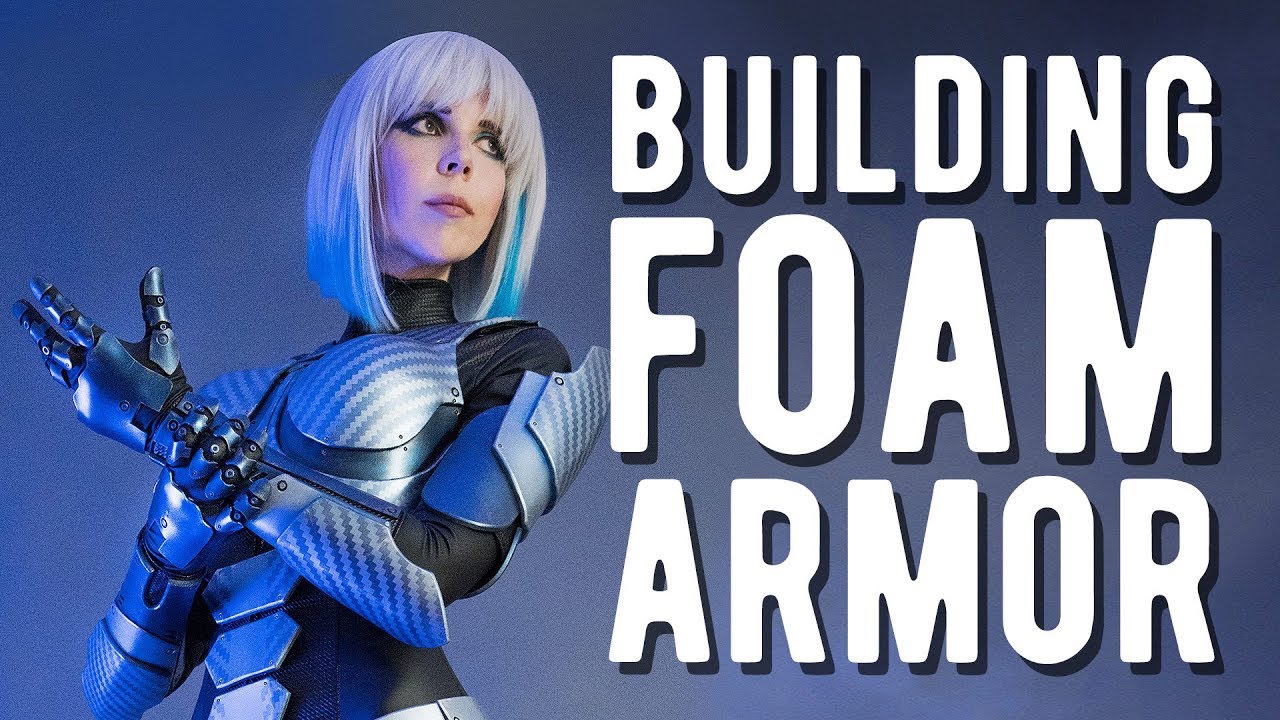The image presents a striking, poster-style advertisement with a gradient background that transitions from dark blue at the top to lighter blue at the bottom. Dominating the right side of the image is a large, white, capitalized font that reads "BUILDING FOAM ARMOR." The figure on the left side is a woman with a futuristic appearance, depicted from the head to the waist. She sports a short platinum bob with bangs and a blue streak. Her makeup is dark and dramatic, enhancing her robotic look.

She is dressed in an elaborate outfit that suggests a blend of comic-con and futuristic robotics, featuring a black leotard beneath metallic armor resembling a chest plate and robot-like gloves. Her posture, with one hand grasping the other, showcases the intricacy of her arm armor. This image likely serves as an advertisement, possibly for a product related to the armor she is wearing.